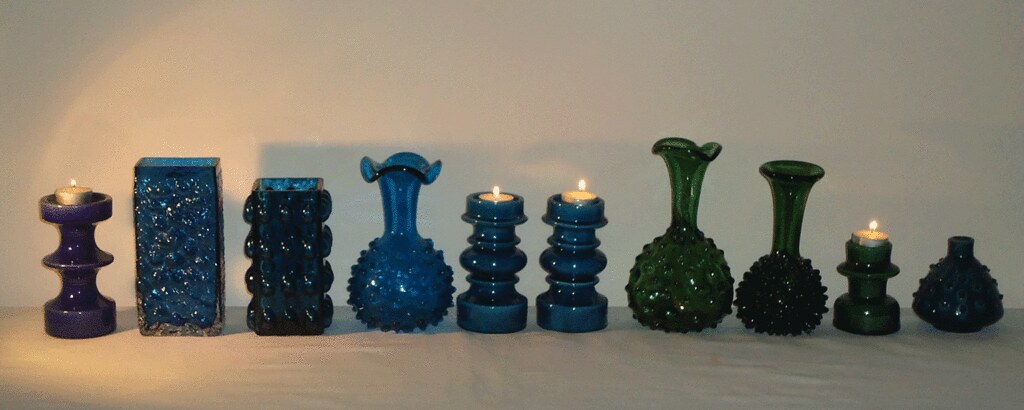This panoramic photograph, about three times wider than it is tall, captures a row of ten vibrant vases and candle holders arranged horizontally against a light brown backdrop, possibly fabric with visible wrinkles. The ambient lighting is warm, creating gentle shadows and adding to the cozy atmosphere. The ornaments are artfully lined up, with colors primarily in purple, blue, and green. 

From left to right, the display begins with a lit, three-tiered candle holder in dark purple, topped with a beige tea light. Next is a square vase adorned with random bubbly textures, followed by a slightly shorter, darker vase with more organized, linear bubbles. Continuing to the right, the scene includes a tall stemmed vase that fans out at the top, featuring a bulbous, bubbly base. 

The centerpieces are two identical candle holders with beige tea lights, resembling the purple one, having rounded, softer tiers. The display continues with a taller vase, characterized by a rippled, green stem and a bubbly bottom, followed by a shorter version with a dramatic, bubble-textured base.

Towards the right end, a shorter candle holder with a lit tea light stands on a simple stem with a large base and circular detailing. The final piece is a small, triangular-shaped vase with a circular opening and small orbs decorating its sides. All the items rest on a beige or white tablecloth, with a beige-colored wall serving as the backdrop, enhancing the colorful and textured display.